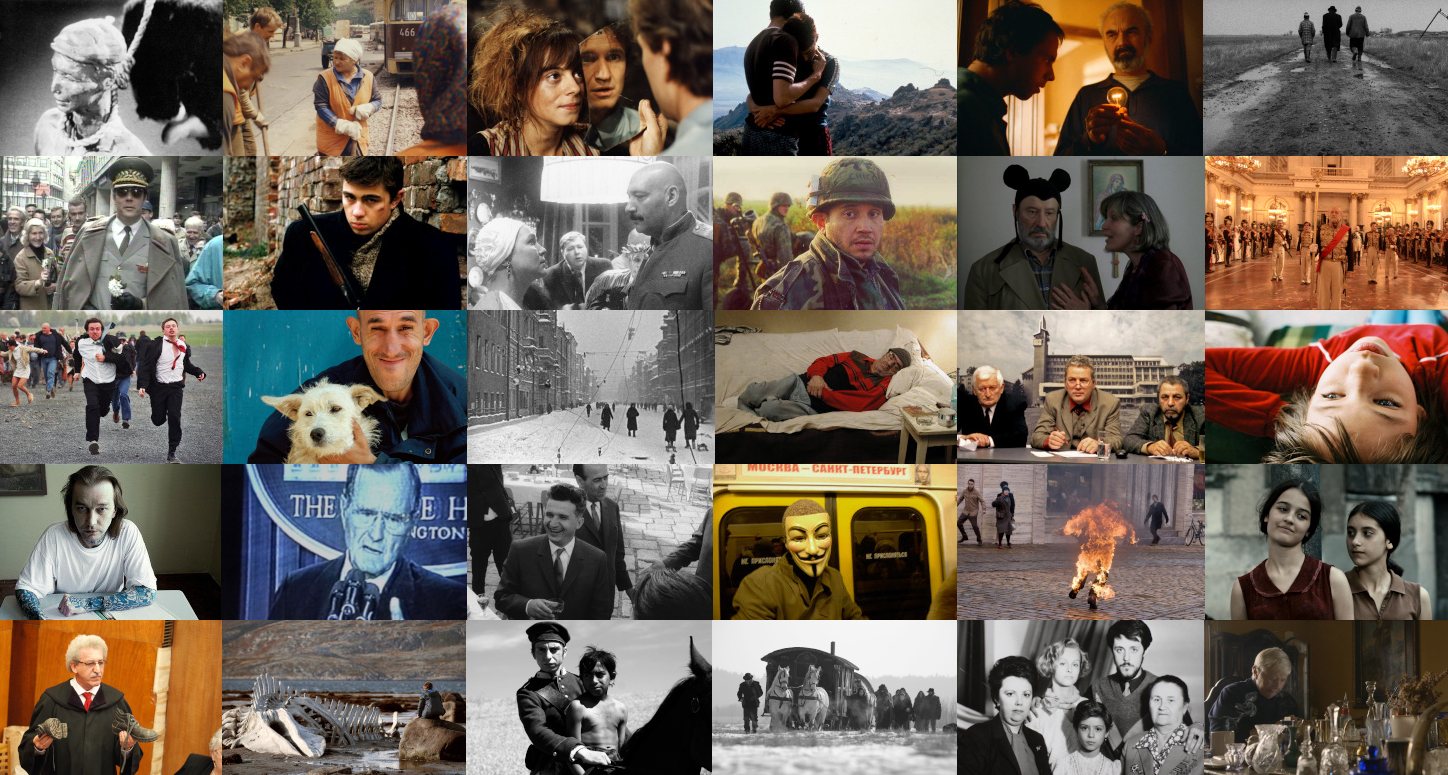This multi-pane collage is an intricate tapestry of individual photographs, blending both black and white and color images, each capturing a unique scene. In the top left, an older woman in a black and white photograph dons a red hat. Below, a busy street scene with three people walking is visible. Nearby, a monochrome image of a soldier looks directly at the camera. On the top right, three people walk down a dirt road in another black and white photo. Directly beneath, a bustling ballroom scene is portrayed.

Towards the center, the yellow doors of a subway frame a person wearing a white mask, exuding an eerie vibe. To the left, a man grins while holding his dog in his lap. Adjacent, a young woman or child is depicted lying on her back, gazing upwards. A man wearing a black judge's robe appears in the lower left corner. Next to him, along the bottom of the collage, lies the skeletal remains of a large whale on a beach, with a monochrome image of a man and a young boy atop a horse near the water to the right.

Further right, a wagon pulled by two white horses appears in a black and white photograph, showing four or five people to the right and one man to the left of the wagon. Next is a family portrait featuring two older women, a young woman, a young bearded man with a mustache, and a small girl in the center. Encompassing diverse activities, the collage also highlights a self-immolating individual engulfed in flames, a mummified figure, workers on a train track, a man looking into a mirror with a woman watching, a couple or siblings embracing, a priest with a light bulb, and a photo of President Bush at a press conference. This rich mosaic of moments, people, and stories offers a vivid and detailed capture of different lives and times.